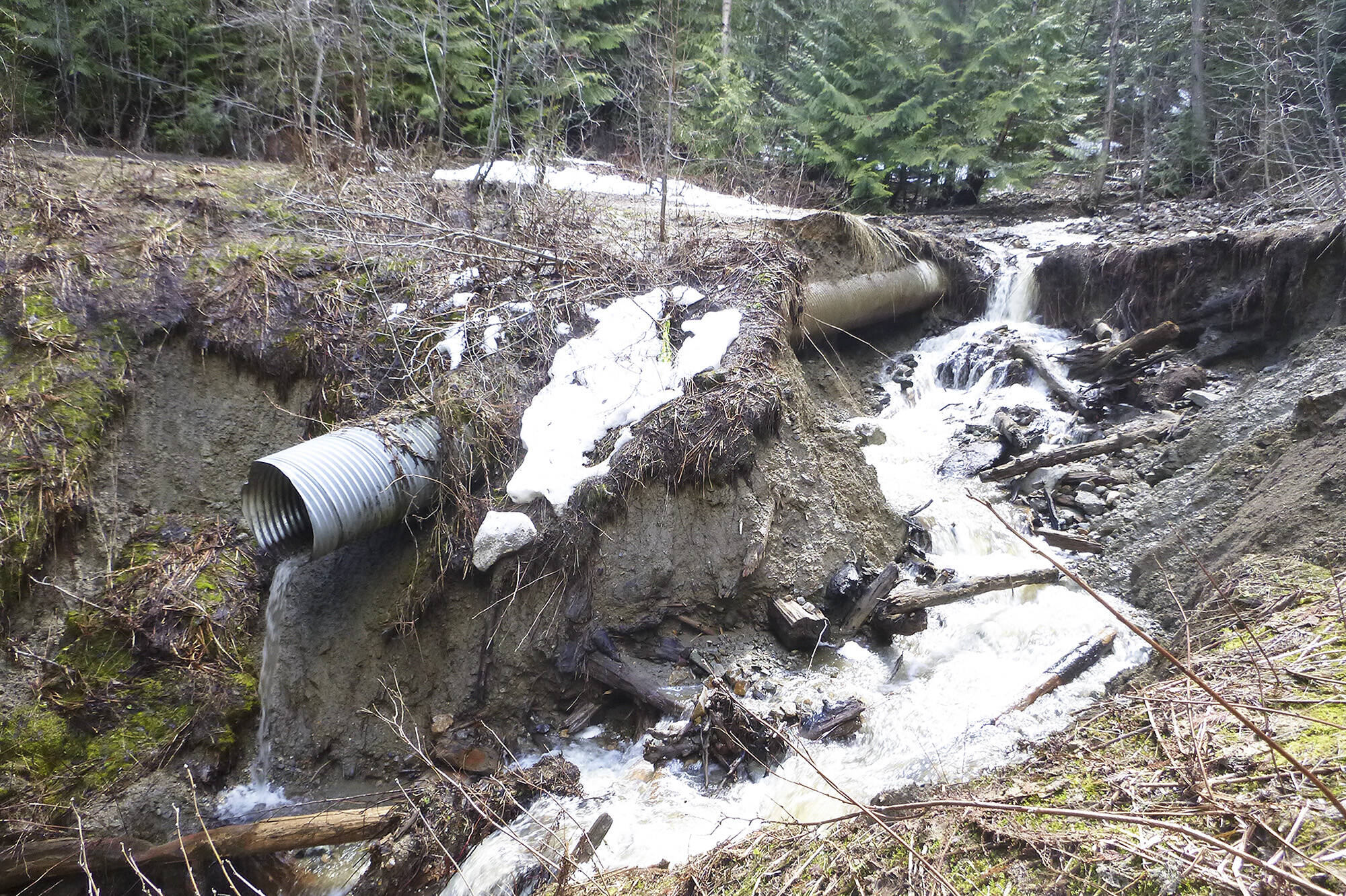The photograph captures a winter or late fall scene in a forested area. Evergreen spruce trees intermingle with barren deciduous trees, reflecting the season. There's a scattered layer of partially melted snow across the ground, suggesting recent thawing. Dominating the scene is a large, silver corrugated metal pipe, partially exposed and emerging from the earth. Water cascades out of this pipe, spilling over a small embankment and merging with a nearby stream that's flowing across the rugged landscape. Twigs and branches are scattered around, adding to the natural, unkempt appearance. The image highlights the natural runoff process in a forest setting, with the human infrastructure of the pipe clearly visible amidst the serene, snowy background.